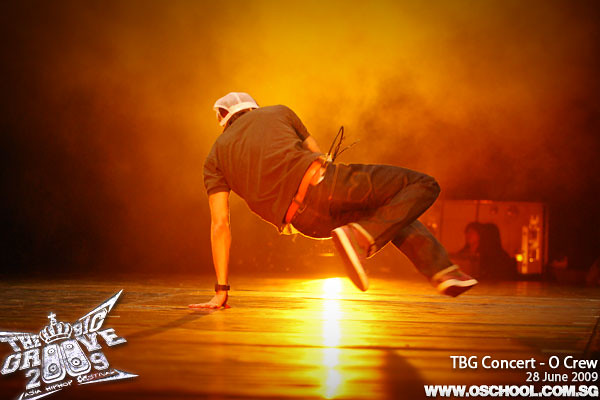In this image from a breakdance performance at "The Groove 2009" during the TBG Concert on June 28, 2009, a dancer is captured in mid-move on a shiny, hard indoor floor. The dancer, positioned at the center of the stage, supports himself with his left hand while his body hovers above the floor. He is dressed in a white, semi-transparent trucker hat, a black shirt, a red belt, and black jeans paired with red and white Nike sneakers. The background includes smoky effects illuminated by an orange light, which add to the dynamic atmosphere. Additional details such as the event name "The Magic Groove 2009 Asia Hip Hop" and the website www.oschool.com.sg are visible at the bottom of the image. To the right, a figure possibly a stage crew member, observes the performance, further indicating the organized, lively concert setting.